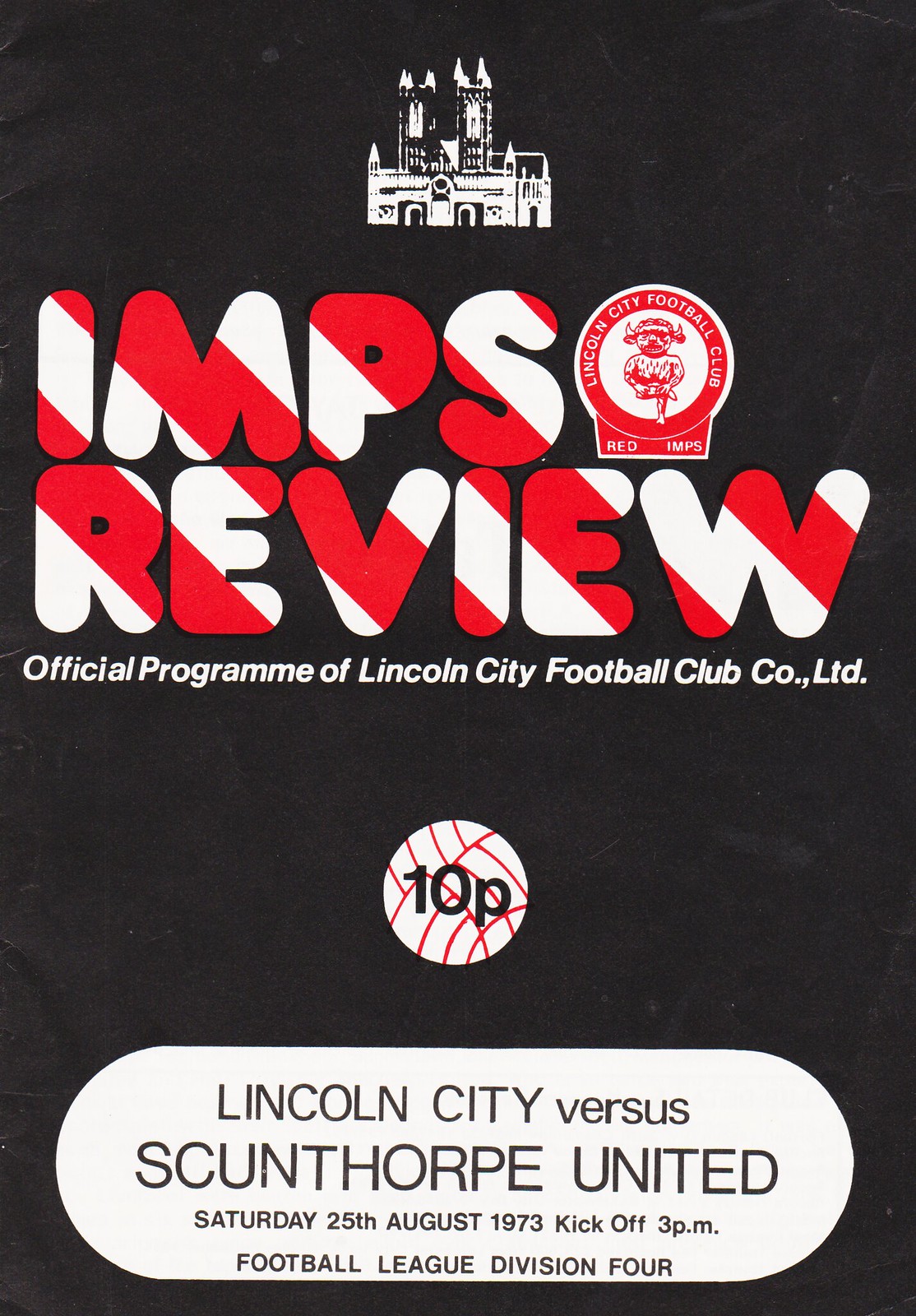The image depicts the cover of a program for a sporting event, specifically a soccer match, featuring Lincoln City Football Club vs. Scunthorpe United on Saturday, August 25, 1973, with kickoff at 3 p.m. The background is black, and the upper part of the cover prominently features a white outline of a castle with two large towers. Beneath this, the title "IMPS Review" appears in extremely bold text with a candy stripe design in red and white, arranged diagonally from top left to bottom right. Below the title, white text reads "Official Program of Lincoln City Football Club Co. Ltd." 

Toward the center of the cover, there is an image of an Imp, a demon-like character standing on one leg with horns protruding from its head. Nearby, there is a circular disk symbol with a red ring and white background, containing the name "Lincoln City Football Club." Further down is a red and white soccer ball logo with black text that reads "10P." At the bottom, within an oval-shaped patch with a white background, black text announces the matchup: "Lincoln City vs. Scunthorpe United." The program also notes that this is part of the Football League Division IV.